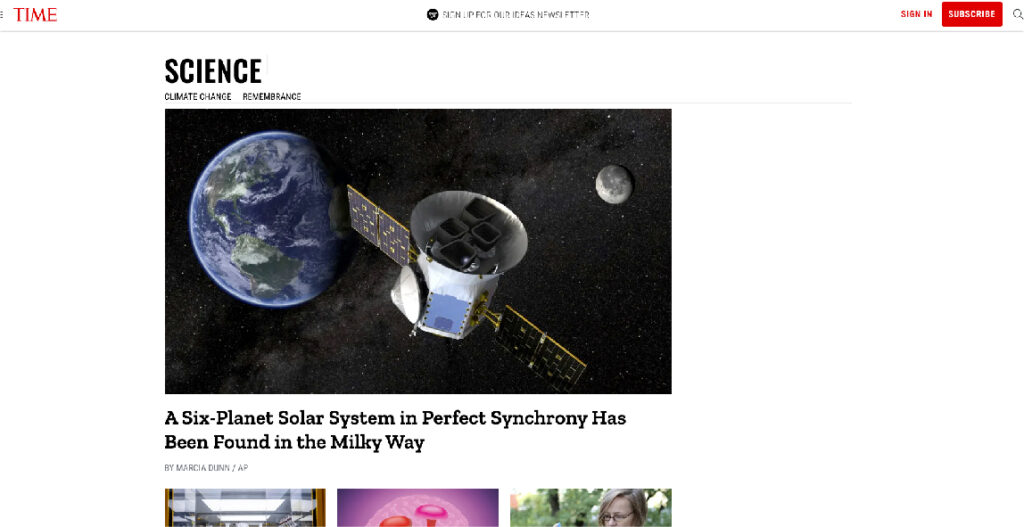This is an updated and detailed caption based on the original description:

---

The screenshot showcases the front page of the Time magazine website. In the top left corner, the iconic Time logo is prominently displayed in its signature red font. In the top right corner, there's a red "Sign In" link followed by a red rectangular "Subscribe" button with white font, and adjacent to it, a small magnifying glass icon indicating a search function.

At the top center of the screenshot, black text—slightly obscured due to the poor quality of the image—appears to prompt users to sign up for the newsletter. Below this text is a large header titled "Science," followed by the subtitle "Climate Change and Remembrance."

Dominating the main section is a large photograph featuring what appears to be a 3D rendered model of a satellite in space. The satellite is set against a backdrop of the dark cosmos, dotted with numerous stars. The Earth can be seen on the left side of the image, while the Moon is visible on the right. Below the photograph, a caption reads: "A six-planet solar system in perfect synchrony has been found in the Milky Way." The byline beneath the title credits Marsha Dunn of the Associated Press (AP).

At the bottom of the image, partially visible, are the tops of three additional photographs, though the majority of these images have been cropped out of the screenshot.

---

This detailed caption captures all the elements described and organizes them cohesively.